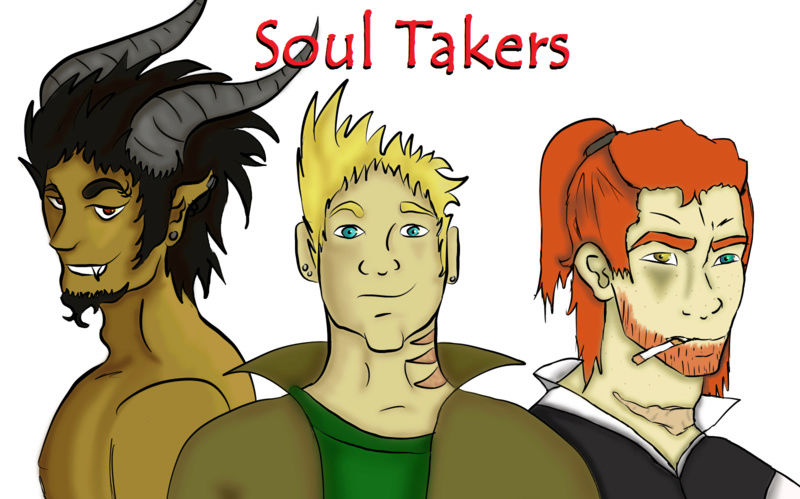This detailed cartoon illustration features three distinct characters sitting together against a white background. The image is titled "Soul Takers," prominently displayed at the top in red ink. 

The character on the left appears to be a demonic or fantasy figure. He has pointed ears, black hair styled haphazardly, and two large, grey horns protruding from his head. His dark skin contrasts with his slanted, red eyes and he wears an arched eyebrow. He also sports a small goatee on his chin and has multiple piercings in his ears, along with an overall malevolent aura.

The central character is a serious-looking man with pointy, spiky blonde hair and blue eyes. He has several earrings in each ear and a noticeable tattoo or scar on his neck. Wearing a green and brown shirt that resembles a cape, he exudes a superhero-like presence.

The character on the right is a red-headed man with his hair tied back in a ponytail. He has a full red beard and is holding a cigarette in his mouth. Notably, he has heterochromatic eyes—one yellowish gold and the other bluish green. His demeanor is somewhat menacing, fitting the overall theme of the "Soul Takers."

Together, these three characters form a motley crew that likely embodies the title’s sinister connotation.